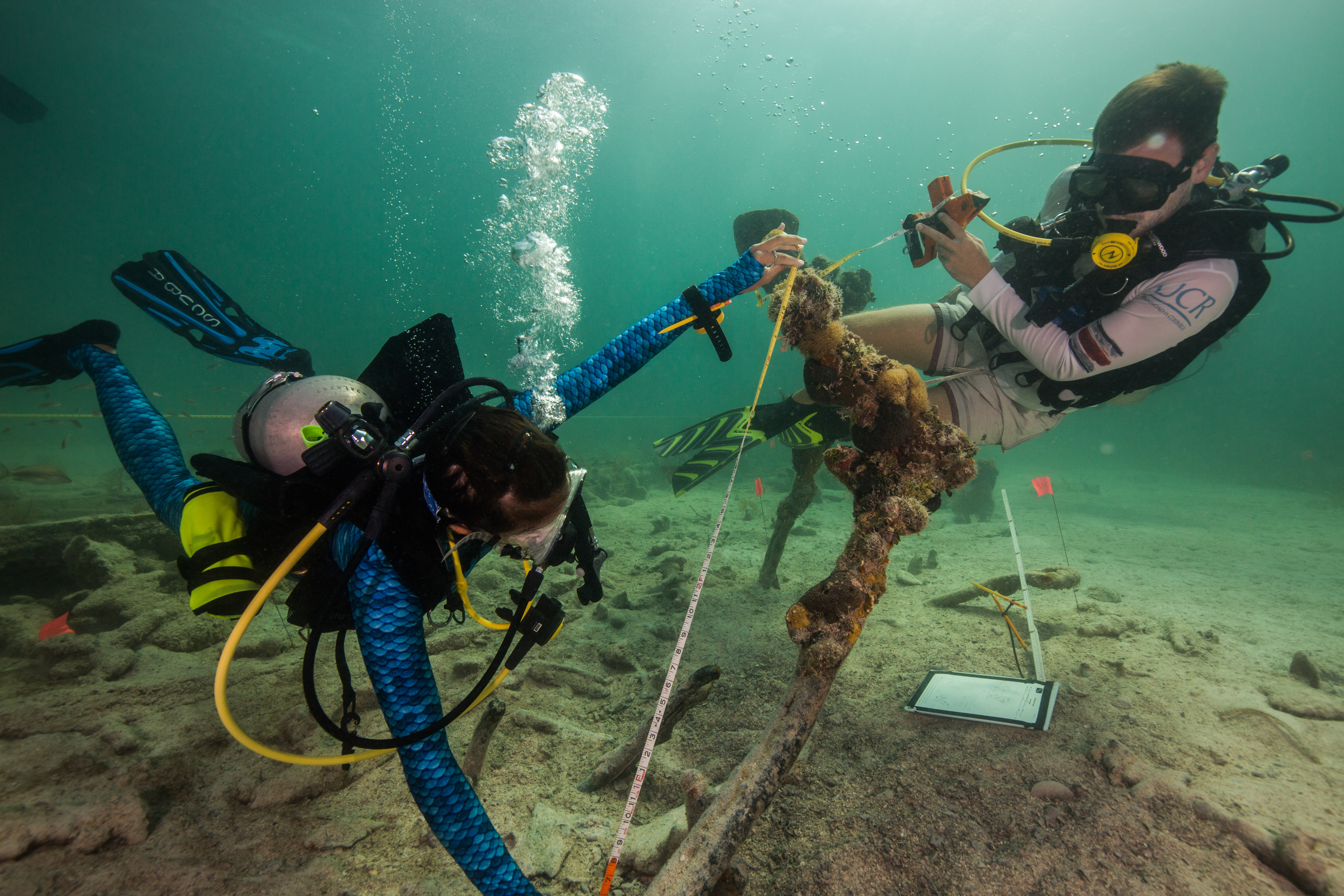This underwater photograph captures two scuba divers exploring the ocean floor. The diver on the left is dressed in a bright blue dive suit with matching fins and has bubbles rising from his head. This diver is extending their arms toward the sea floor, possibly indicating engagement with an object there. Speculation suggests that this diver might be a woman, inferred from the potential presence of hair barrettes.

The diver on the right is wearing light tan shorts, a long-sleeve light-colored shirt, and a dark vest, equipped with an extensive-looking scuba tank system, as seen from the tubes and tank emerging from his back. This diver appears to be photographing their companion, contributing to the cloud of bubbles in the scene.

The ocean floor, primarily sandy, features a few notable objects. Below the right diver, there is a rectangle-shaped item resembling a clipboard or an electronic tablet, suggesting the presence of research equipment. Additionally, the sandy surface contains a multicolored, thick stick-like object, described as having brown, red, and yellow hues and vaguely resembling a gun in shape, though its exact purpose remains unclear. The surrounding water is greenish, with sunlight filtering through, encapsulating the divers' activity in a bright, immersive, and visually striking underwater environment.